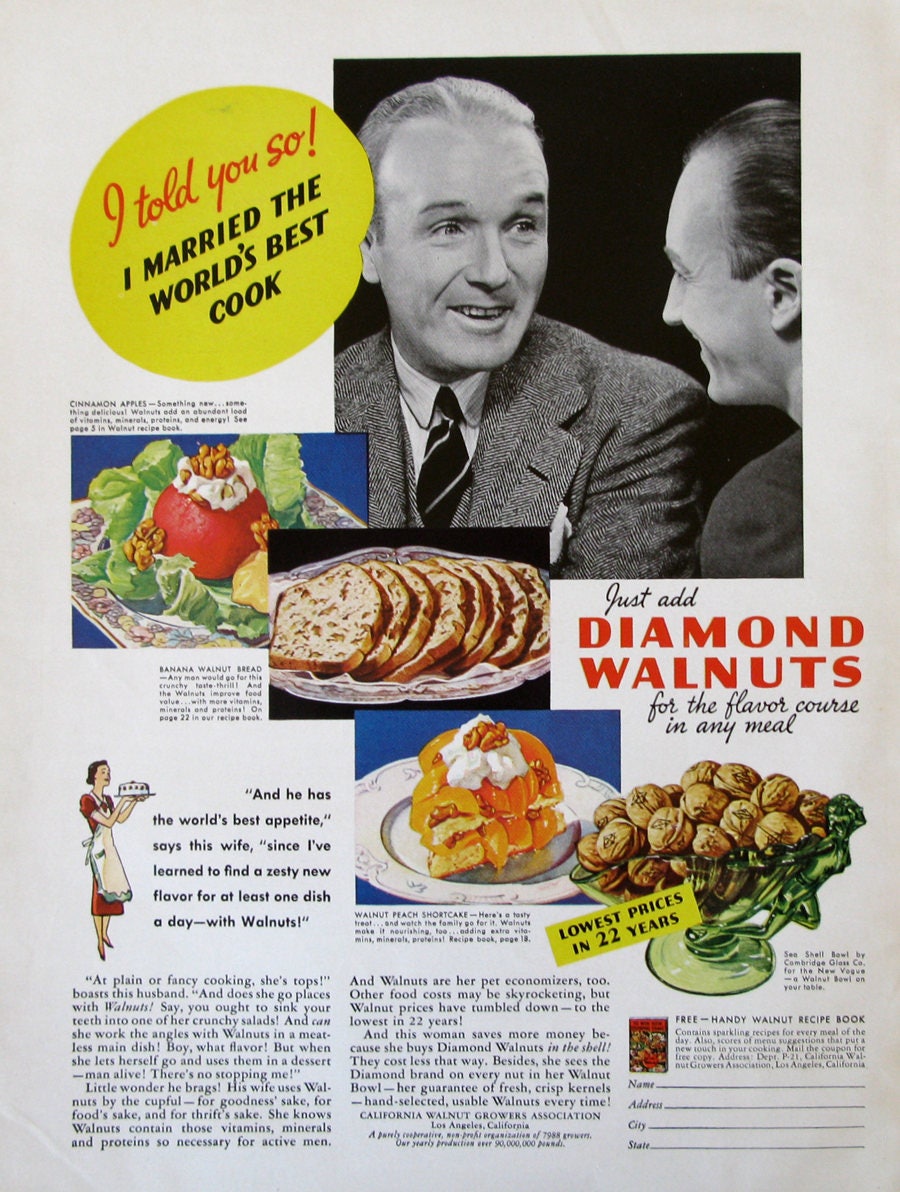This image is an advertisement from a vintage magazine, likely from the 1940s or 1950s, promoting a free walnut recipe book. It features multiple visuals centered around walnuts and their culinary uses. In the top right corner, there's a photograph of two men engaged in conversation; the man on the left, dressed in a gray tweed suit with a white collared shirt and striped tie, is speaking animatedly to the man on the right, who has slicked-back black hair and is wearing a sport jacket. A caption above them reads, "I told you so, I married the world's best cook."

Adjacent to the photograph, the ad highlights various walnut-based dishes. Below the men, there's an image of an apple coated in chopped walnuts with cinnamon, described as "something new, something delicious." Further down, a picture of banana walnut bread is showcased, suggesting it would be a "crunchy taste thrill" and noting that walnuts enhance its nutritional value with added vitamins and minerals. Another inset features a glass bowl of walnuts next to a cake topped with whipped cream and a single walnut, promoting the idea to "just add Diamond Walnuts for the flavor course in any meal." The top left of the page features a yellow circle with the text, "See page 5 in walnut recipe book," guiding readers on where to find more delicious walnut recipes. Overall, the advertisement emphasizes the culinary benefits and versatility of walnuts.